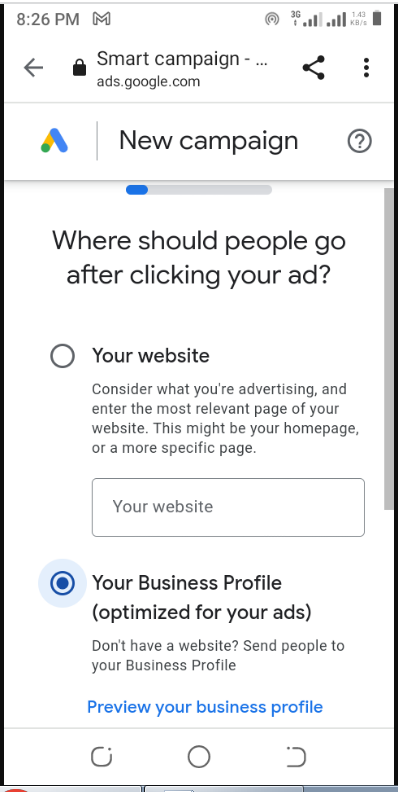A close-up image of a smartphone screen displaying the home screen at 8:26 p.m. is depicted. At the top, the screen showcases the current time along with clear icons for Google Maps, Wi-Fi signal, and battery life. Just beneath these icons, an advertisement for Google's Smart Campaign is prominently visible. The ad, labeled by "ads.google," prompts the user to start a "New Campaign." Directly below the main message, it asks, "Where should people go after clicking your ad?" and presents two actionable buttons: one labeled "Your Website" and the other "Your Business Profile Optimized for Your Ads." The overall image provides a detailed snapshot of a typical user's mobile interface while engaging with Google's ad platform.